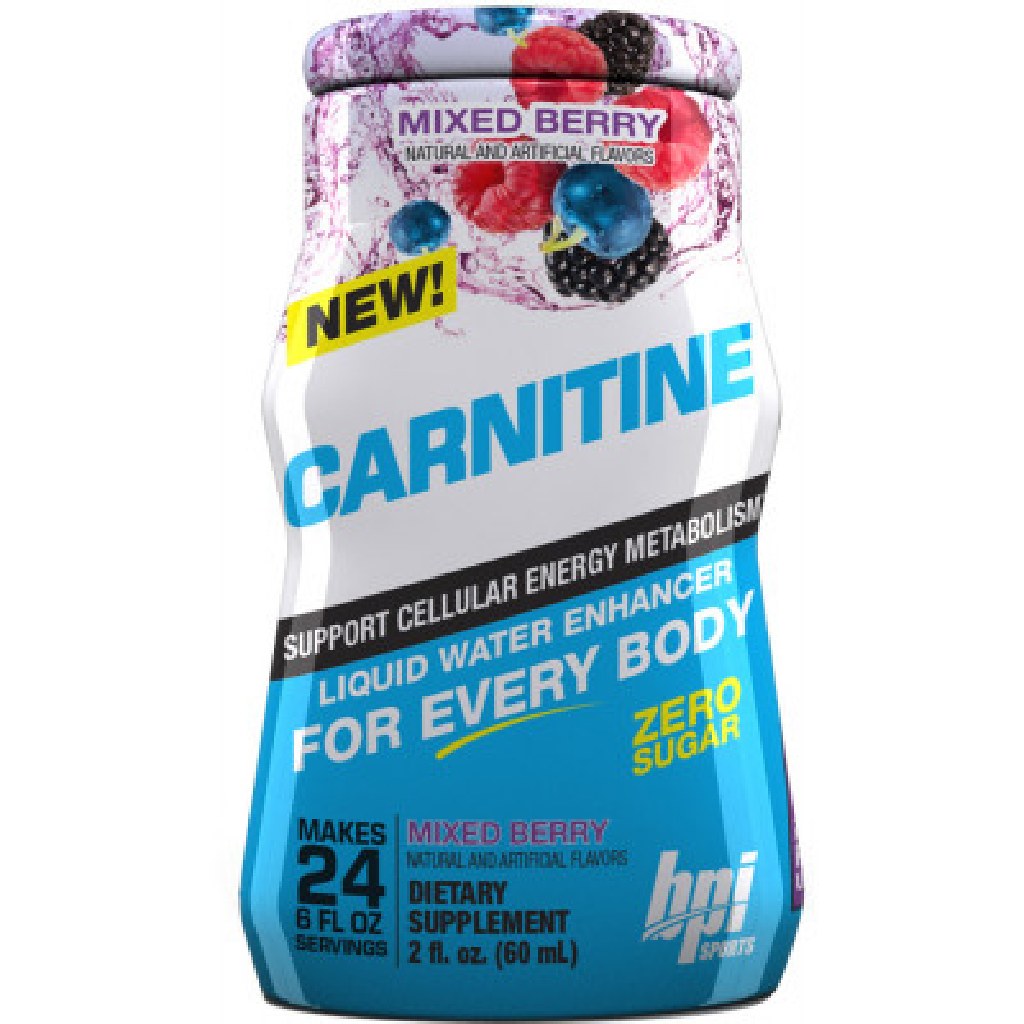The image is an up-close shot of a plastic dietary supplement container from the brand BPI Sports. The bottle, which is white and blue, is decorated at the top with images of raspberries, blackberries, and blueberries, and features a design of liquid pouring into a glass. The product label prominently states "Mixed Berry" in purple font and mentions it contains both natural and artificial flavors. There's a yellow stamp indicating it's a "new" product, and the name "Carnitine" is highlighted in bold blue letters. The product claims to support cellular energy metabolism and serves as a liquid water enhancer with zero sugar, making 24 servings of six fluid ounces each. The bottom of the bottle reiterates the claims, with text in white on a blue background, and additional details including "dietary supplement," "supports cellular energy metabolism," "new carnitine," and the specific measurements of two fluid ounces (60 milliliters). The bottle design tapers in the middle and widens slightly before narrowing again towards the top.